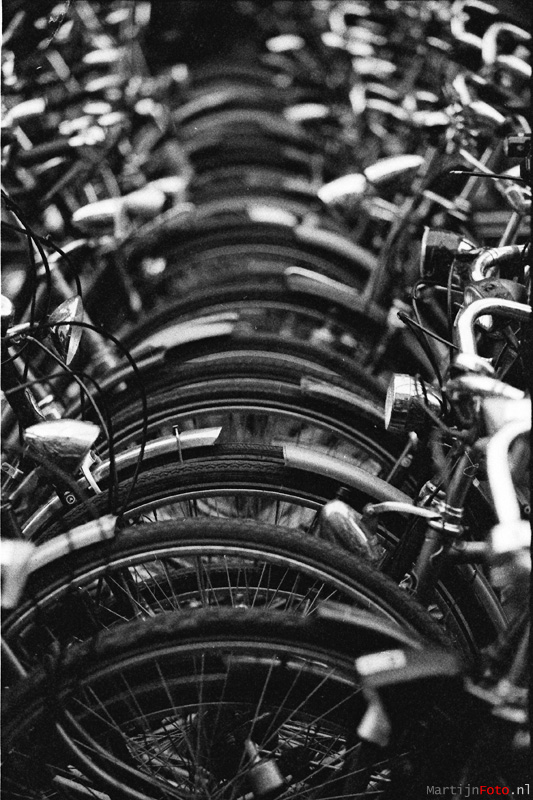This black and white photograph depicts a tightly packed line of bicycles extending from the bottom of the frame to the blurred background, creating a repetitive and rhythmic pattern of overlapping components. The bicycles are arranged in alternating racks on either side, ensuring their handlebars do not touch while allowing them to be parked extremely close together. Visible details include the black tires with notable treads, white fenders, and an array of spokes. The photo is rectangular in shape and features text at the bottom: "M-A-R-T-I-J-N" in gray, "F-O-T-O" in red, and ".N-L" in white. While the handlebars and other bicycle parts are partially visible, the primary focus remains on the wheel formations that dominate the scene, highlighting the dense configuration of the bicycles parked in this organized yet visually intricate manner.